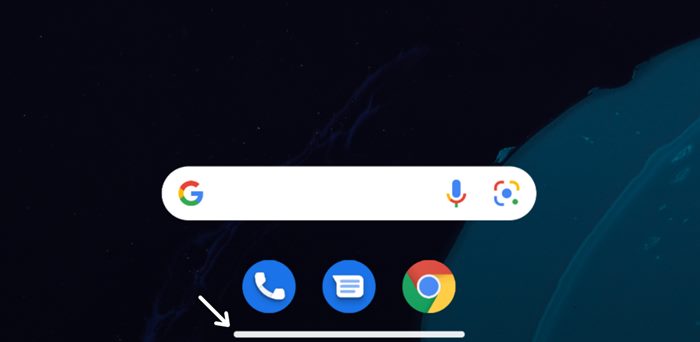The image features a Google search bar prominently in the center, set against a bluish-black background that resembles a nighttime scene. A bluish circle is visible emerging from the bottom right corner. The search bar itself is white, with the multicolored Google logo ("G") on the left side, displaying red, yellow, green, and blue hues. To the right within the search bar, there are two icons: a microphone icon and a camera icon. Below the Google search bar, there are three additional icons: a phone icon, a messaging icon, and the Google Chrome icon. Further down, a thin white line with an arrow is visible, completing the layout of the image.